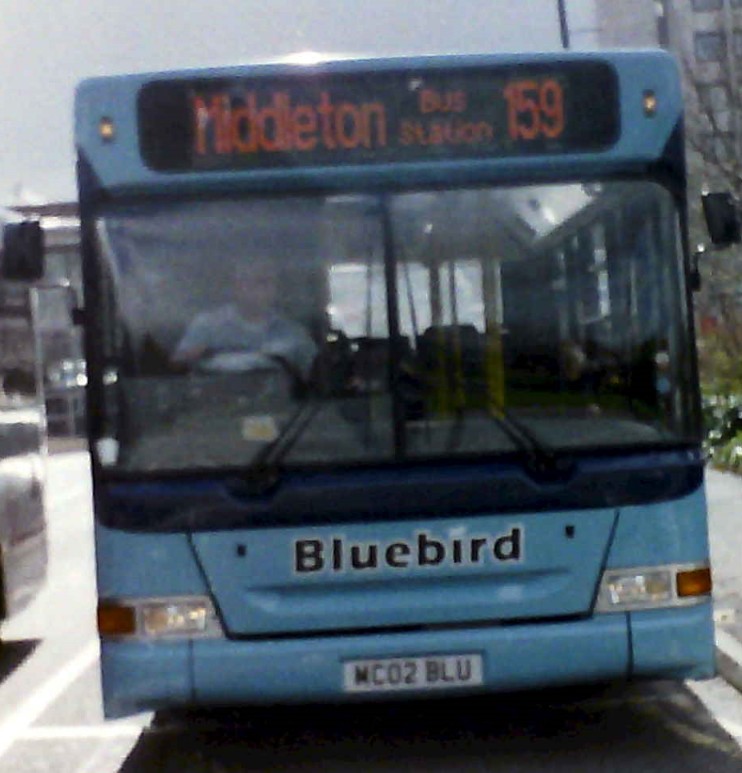This photograph depicts the front of a blue city bus in a somewhat blurry and grainy image, taken from a position directly in front of the vehicle. The bus prominently fills approximately 80-90% of the frame. It features a large windshield with small headlights below. The bus displays the destination "Middleton Bus Station 159" in orange letters on a black sign at the top front. Below this, the name "Bluebird" is printed in black text, and its license plate reads MC02BLU. The driver, clothed in a blue shirt, is visible through the large front window. This right-hand drive bus appears to be situated on a street during daytime, with adjacent buildings visible in the background on the top right, a car next to it, and trees along with a high-rise building in the distance.